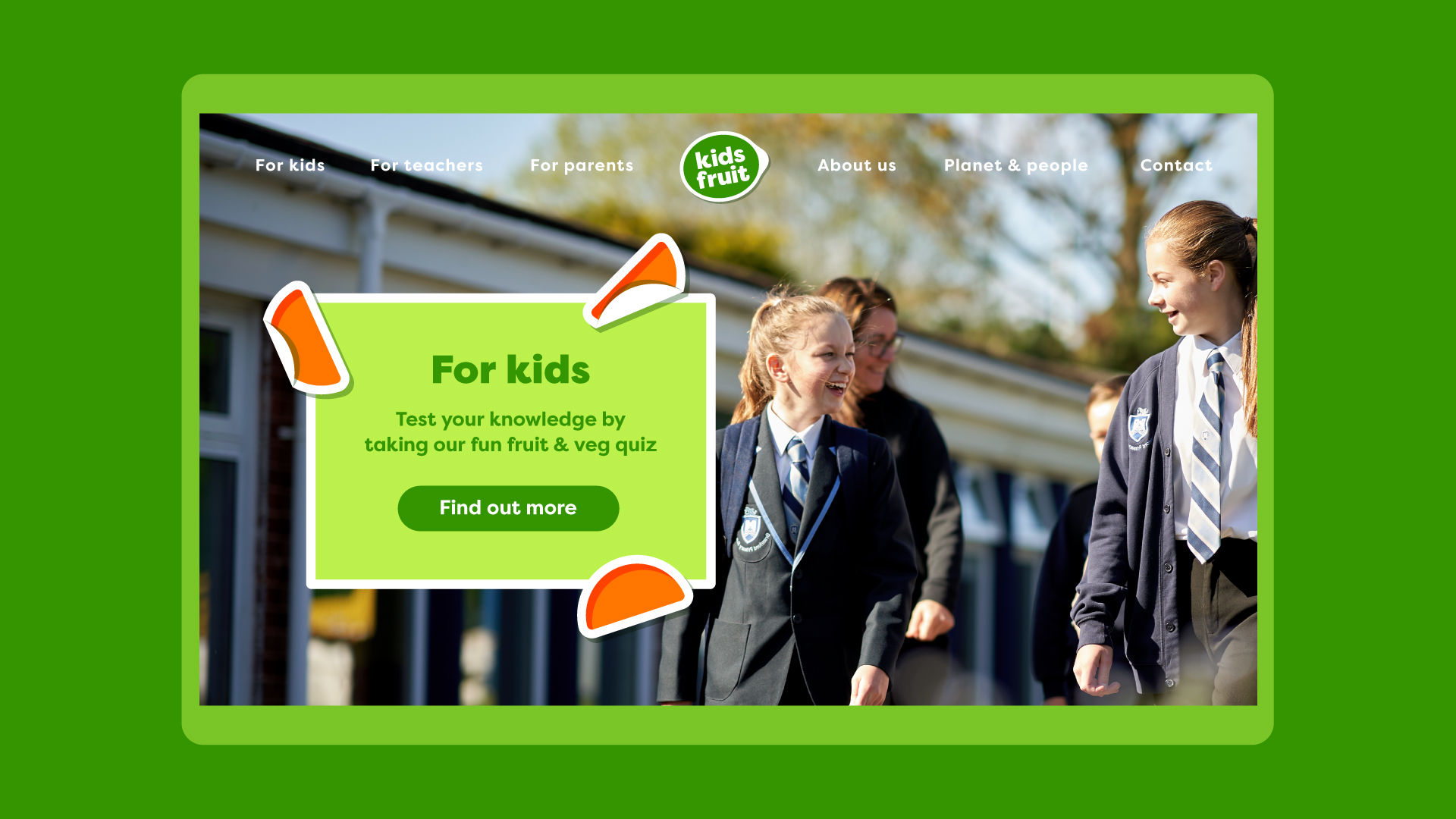In the image, a lime green website design features a central photograph of a group of schoolgirls dressed in private school uniforms. The uniforms consist of blazers, sweaters, black pants, and striped navy and gray ties. The students, all with ponytails, are of various heights and are engaged in conversation as they walk in front of a large school building. A prominent tree stands behind the school, adding greenery to the scene. 

At the top of the website, a bold green header with a white liner displays the text "Kids Fruit" along with navigation options, including "For kids," "For teachers," "For parents," "About us," "Planet and people," and "Contact." 

Within the image, there is a lime green box that features an almost circular design element with orange half-circles edged in white. The box invites users with the prompt, "For kids, test your knowledge by taking our fun fruit and veg quiz," and includes a darker green box with the call-to-action "Find out more."